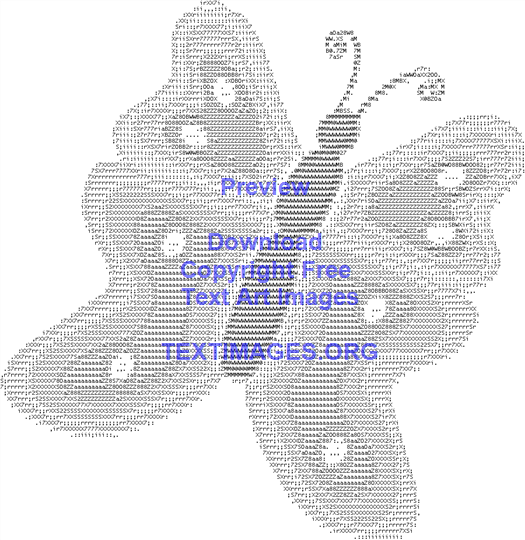The image depicts a pixelated gray butterfly created using small letters and numbers, emblazoned with a light purple watermark that reads, "Preview, Download, Copyright-Free Text Art Images" in a sans serif font. Positioned diagonally, the butterfly is centrally placed with its body and long curly antennae extending to the top right. The top left wing points upward to the top left, while the lower right wing extends to the bottom right. The butterfly's upper wings feature four white oval dots, mirrored by another set of four on its larger lower wings. The watermark includes the website URL, "textimages.org" at the bottom. The setting gives the impression of an advertisement for a website offering downloadable text art images, including this butterfly.